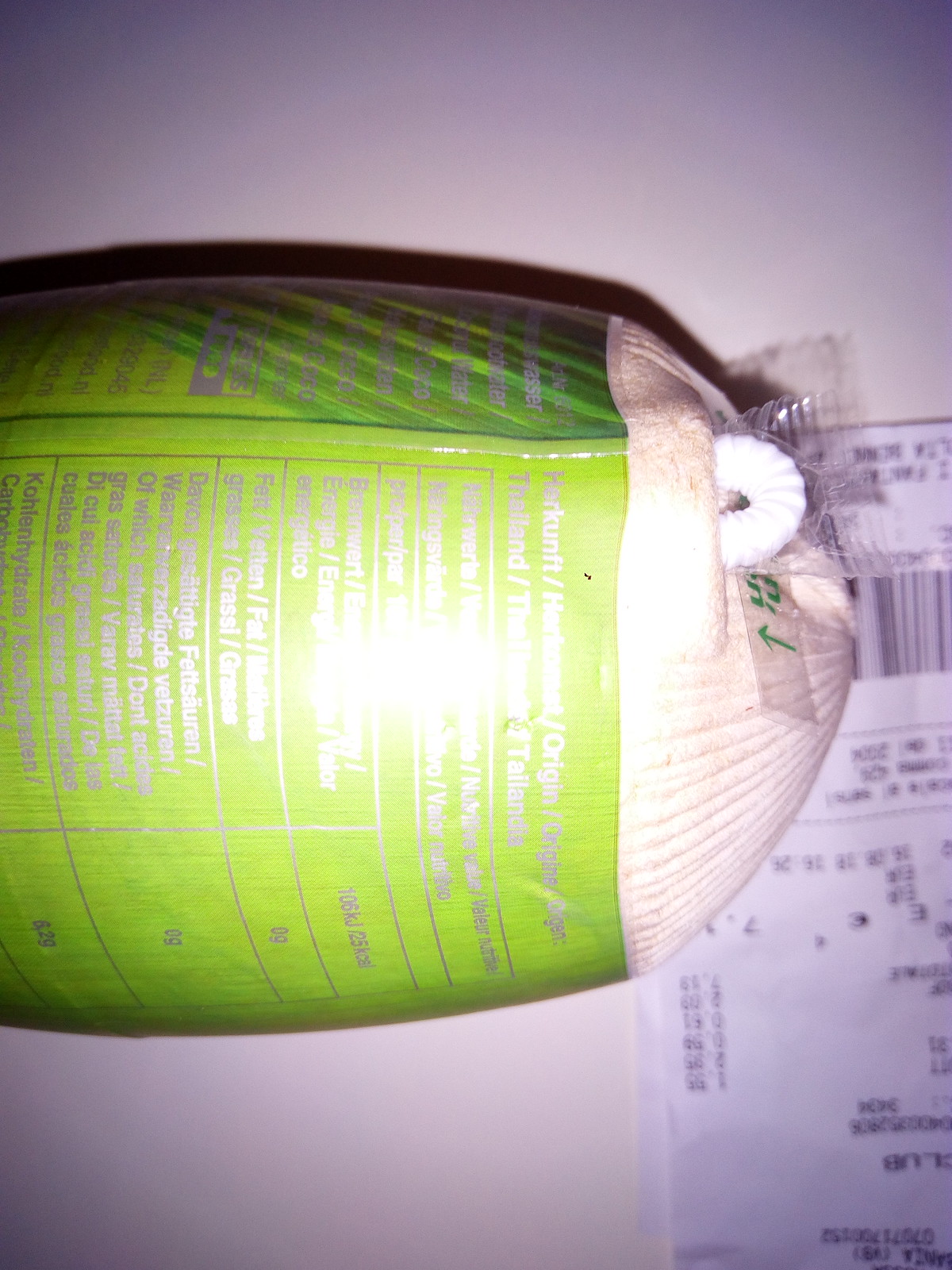This is a close-up photograph of an unknown item, potentially a hammock or a sleeping bag, encased in a storage bag. The bag features a green label adorned with text that is difficult to decipher, possibly due to the reflective glare from the camera's flash. The text might not even be in English. On the right side of the bag, a white piece of fabric is visible, with a rope end protruding from it. The photograph is taken on a white background, and a paper receipt is visible to the right side of the image, adding an additional element of context.